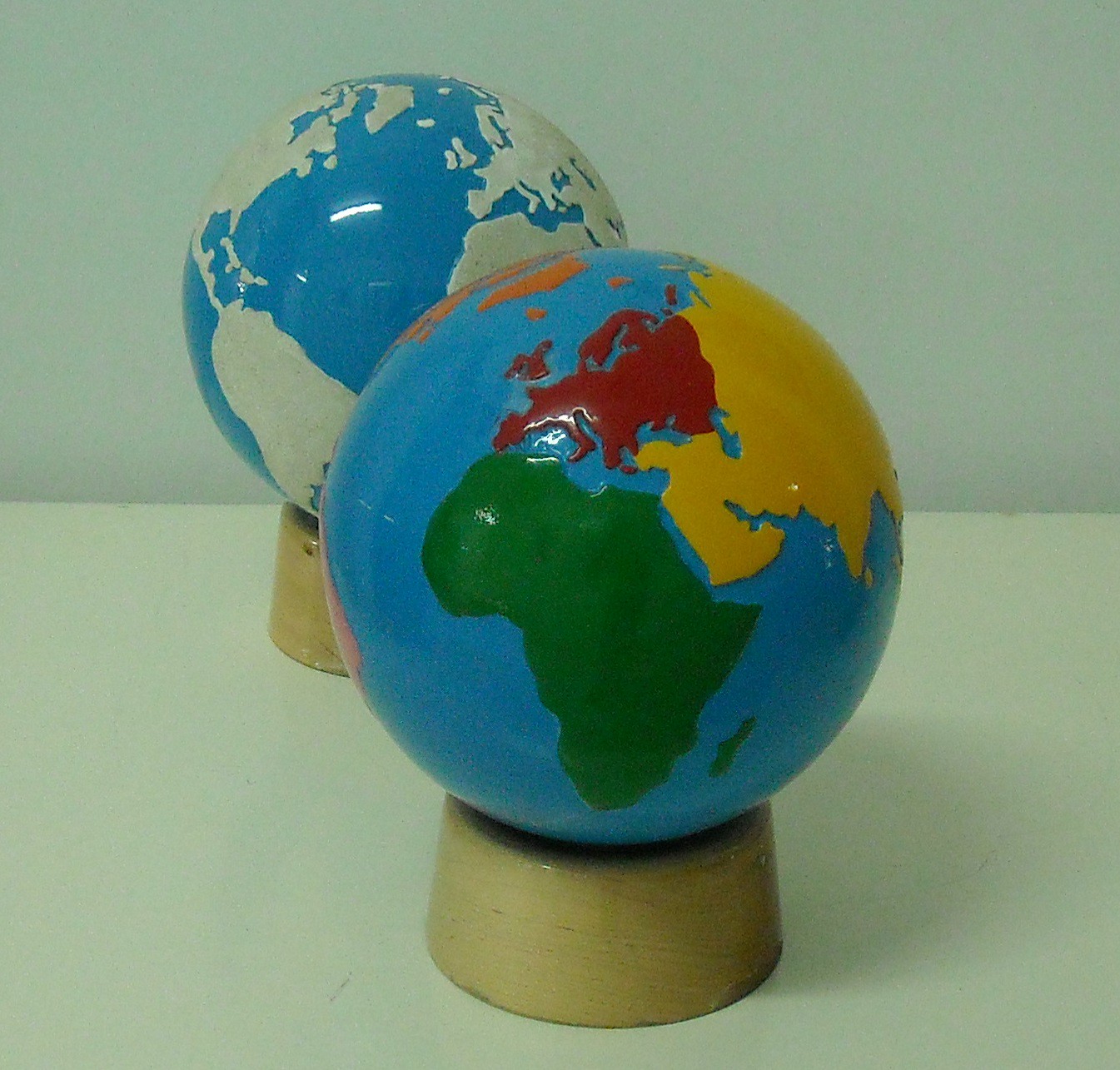This color photograph, likely taken in poor indoor lighting or with a dark greyish filter, depicts two model globes of the Earth on light brown wooden bases. The primary globe, positioned centrally and occupying about three-quarters of the image, showcases Europe, Africa, and Asia in vibrant hues: Europe in red, Africa in green, Asia in yellow, and Iceland and Greenland in orange, all set against bright blue oceans. It's placed slightly towards the bottom right. The secondary globe, slightly behind and to the left, displays a rotated view focusing on the Atlantic Ocean and parts of North and South America; the continents appear in grey or white, also against blue waters. Both globes exhibit a shiny finish. The background and surface have a grey, muted greenish tinge, likely due to the dim lighting, with a small light source casting a slight shadow of the closest globe to the bottom right, indicating illumination from the left.